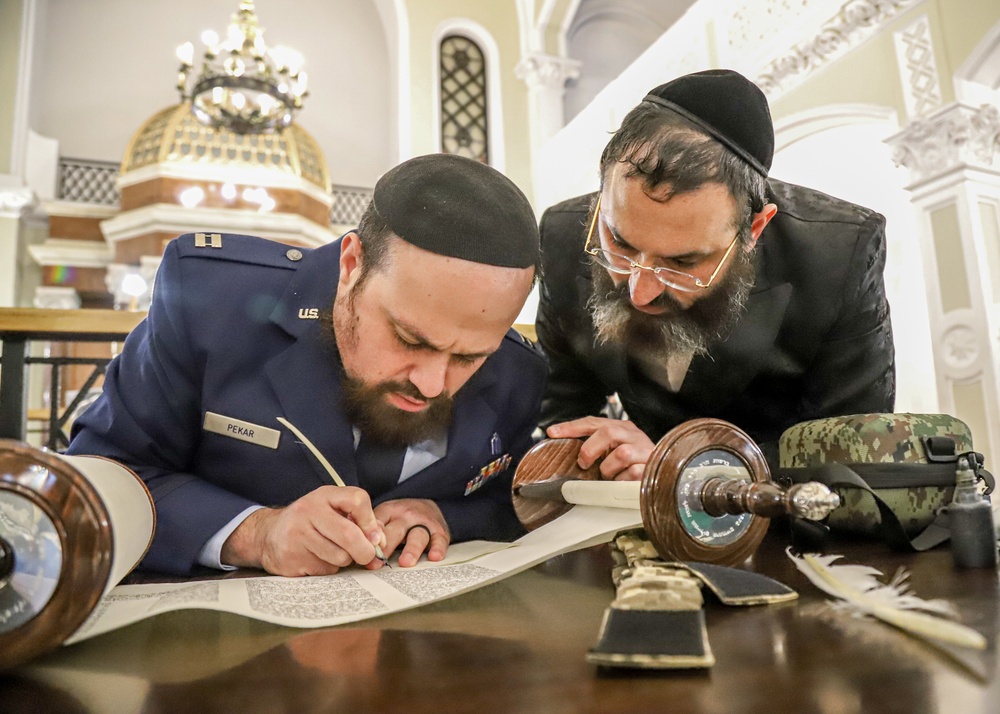The image depicts two bearded men inside a large, prestigious building with white and tan walls, likely a synagogue or library, featuring an elegant chandelier hanging from a tall roof. Both men are adorned with traditional Jewish yarmulkes. The man on the left, identified as "Pekar" from a name patch on his dark blue military uniform, is seated at a dark brown wooden table, decorated with medals of honor suggesting significant accomplishments. He is writing on a large, rolled-out scroll using a pen, possibly in an old-fashioned scribe manner. The man on the right, dressed entirely in black with glasses and a mixed brown-black beard, appears to be a rabbi leaning over Pekar's shoulder, observing the writing process. Other items on the table include a camouflage-colored backpack and an army container, possibly for water or tools. The setting is well-lit, indicating the photograph was taken during the daytime.